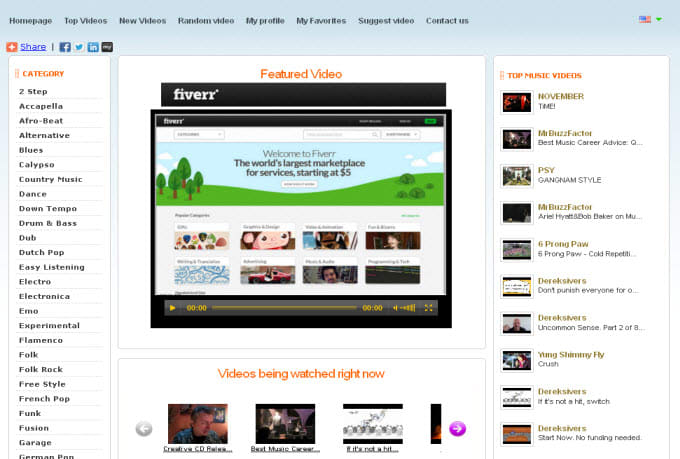This screenshot image appears to be from the Fiverr website. At the top of the screen, there are various navigational tabs including 'Homepage,' 'Top Videos,' 'New Videos,' 'Random Video,' 'My Profile,' 'My Favorites,' 'Suggest Video,' and 'Contact Us.' Directly beneath these tabs, you can see social media icons for sharing content, specifically for Facebook, Twitter, LinkedIn, and one other indistinct icon.

On the left-hand side, there is a list of categories presented in alphabetical order. These categories range from diverse musical genres such as Two-Step, Acapella, Afrobeat, Alternative, Blues, Calypso, Country Music, Dance, Down-Tempo, Drum and Bass, Dub, Dutch Pop, Easy Listening, Electro, Electronica, Emo, Experimental, Flamenco, Folk, Folk Back, Freestyle, French Pop, Punk, Fusion, Garage, and German Pop. The list appears to be extensive, but only a portion is visible in the screenshot.

Occupying the main section of the screenshot, there is a black banner at the top labeled 'Featured Video.' Below this banner, to the left, is the Fiverr logo. Beneath the logo, there is a video thumbnail which indicates that users can play videos directly on the Fiverr website. The overall layout seems to be user-friendly, providing easy navigation through various categories and options.